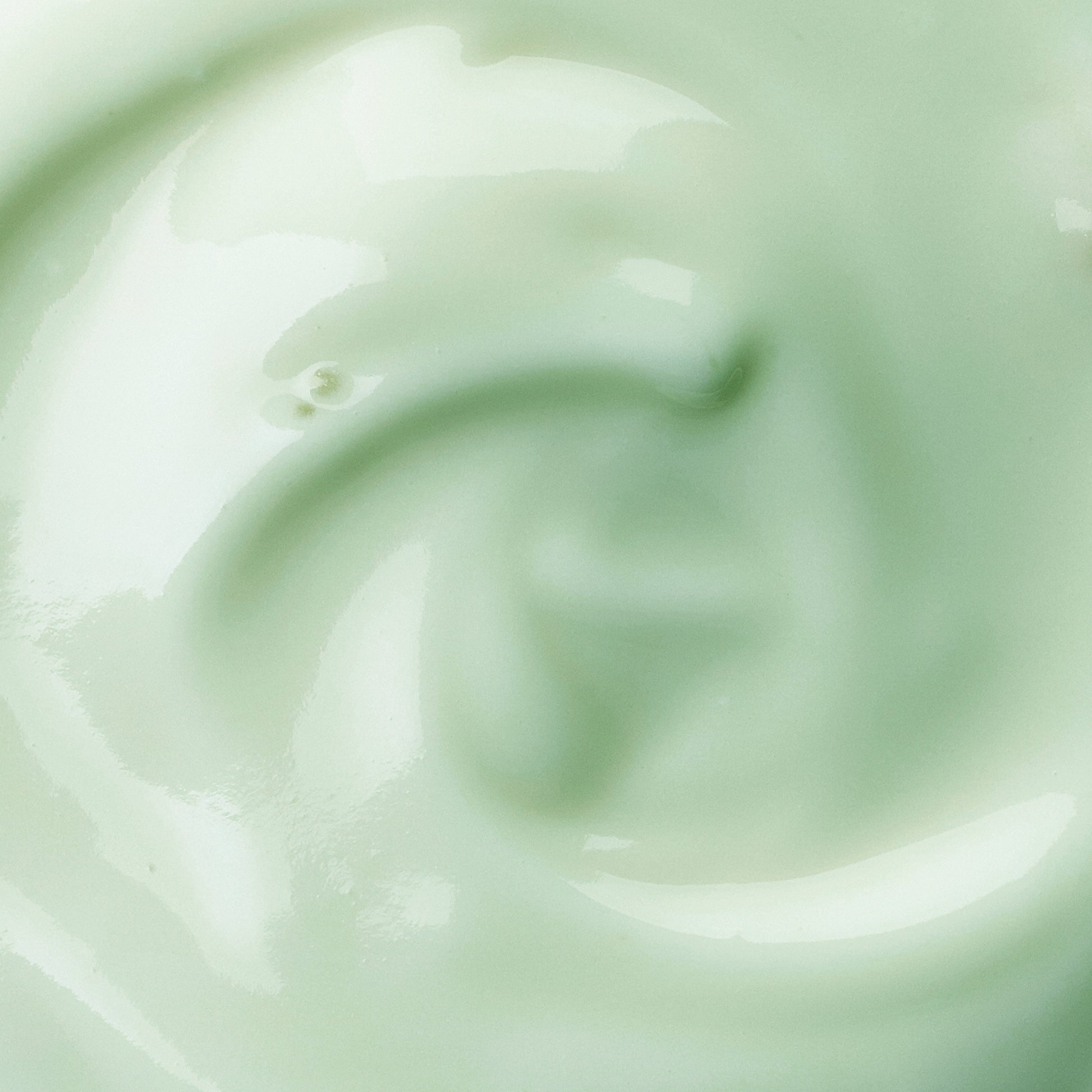The image appears to depict a top-down view of a creamy, greenish-white substance, likely resembling homemade yogurt or a gel-like material. The primary hues are varying shades of white and light green, with the surface exhibiting a reflective sheen that catches the light. The substance fills the entire frame, obscuring any details that might indicate the type of container it is in or the surroundings. The texture is smooth with distinct swirling patterns that appear to have been created by a clockwise, circular motion. These swirls originate from various points: one starts from the bottom right, curving up and to the left, while another begins from the middle bottom, arching up towards the center and then to the right. There are also subtle ripples, particularly two prominent small air bubbles near the center swirl, where the bubble on the right is notably larger than the one on the left. Overall, the image evokes a sense of fluid movement and creamy consistency without any distinguishable context to reveal the time of day or setting.